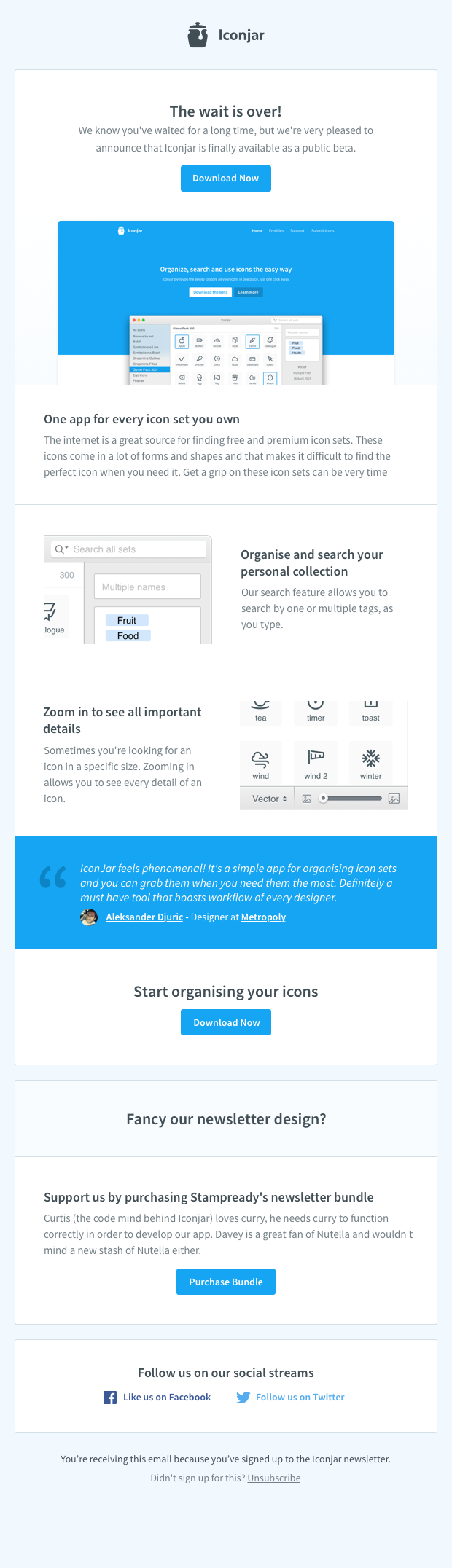This is an image of the Icon Jar newsletter, showcasing the features and benefits of the Icon Jar application in a visually appealing layout.

The background of the newsletter is a light blue, providing a calm and inviting atmosphere. At the very top, the title "Icon Jar" is displayed in dark grey, accompanied by an image of a jar.

Inside this blue window, a white section contains detailed information about the Icon Jar website. At the top of this section, a prominent headline announces: "The wait is over! We know you've waited for a long time, but we're very pleased to announce that Icon Jar is finally available as a public beta." Beneath this announcement is a blue "Download Now" button.

A screenshot of the Icon Jar website illustrates the application's interface and features, showcasing various icons. Following the visual, a headline states: "One app for every icon set you own," emphasizing the versatility of the application. Another headline reads: "Organize and search your personal collection," paired with an image demonstrating how icons are organized, including categories like "multiple names," "fruit," and "food."

The final headline, "Zoom in to see all important details," is supported by an image depicting the zoom-in feature for viewing icons in greater detail.

At the bottom of this section, a testimonial from Alexander Jurek is displayed: "Icon Jar feels phenomenal. It is a simple app for organizing icon sets, and you can grab them when you need them. Definitely a must-have tool that boosts the workflow of every designer."

The bottom of the newsletter reads: "Start organizing your icons. Download now." A smaller section underneath promotes the "Stamp Ready’s Newsletter Bundle." A blue button here encourages readers to "Purchase Bundle."

In summary, this detailed and structured image provides comprehensive insight into the features and benefits of Icon Jar through its newsletter.